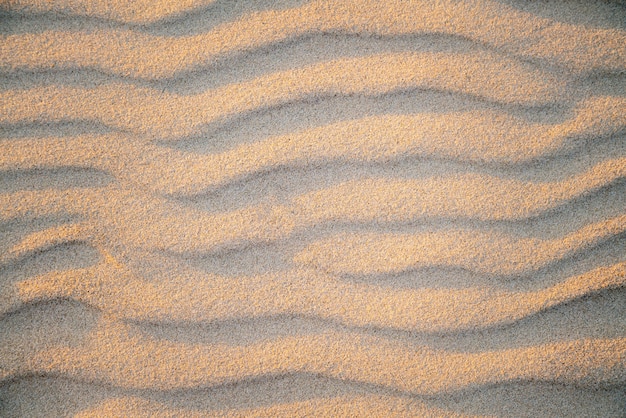This photograph, likely taken outdoors, captures a striking horizontal rectangle scene featuring a series of raked sand layers. These layers create a distinct wave pattern, with each successive wave slightly elevated above the previous one. The image showcases about seven or eight rows, extending predominantly from the left edge to the right, though one wave in the center-right notably tapers off midway. The sands display shadows underneath the crests, accentuating the wave effect. The beige-yellow sand, interspersed with hints of red and orange dust, presents a color palette that shifts to pinkish and purplish tones. The fine grains and the curving lines, shaped by the wind, give the appearance of ripples or steps, adding depth and texture to the photograph.